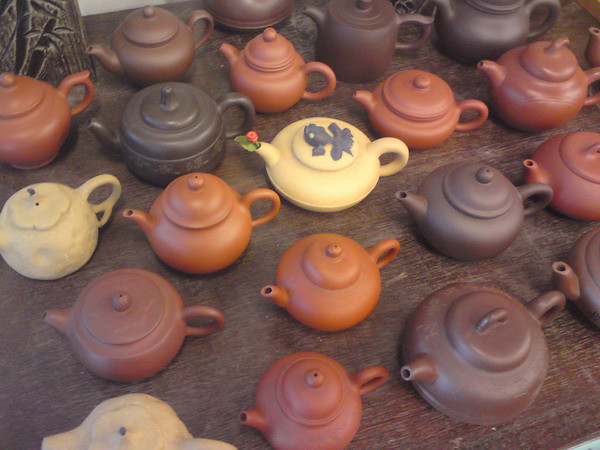The photograph captures an overhead view of a slightly worn, deep brown wooden table, allowing the grain patterns and scratches to show through. The table is meticulously covered with rows of ceramic teapots of various sizes, shapes, and colors. The teapots predominantly feature earthy tones, including at least three different shades of brown, with a few muted yellow, orange, and red ones adding a touch of vibrant contrast. Each teapot has its handle to the right and spout to the left, forming a uniform pattern. Among them, a yellow teapot in the center stands out due to a sculpted gray clay flower and a tiny red rose with a leaf detail on its spout, and some dark brown stylized detailing on its handle.